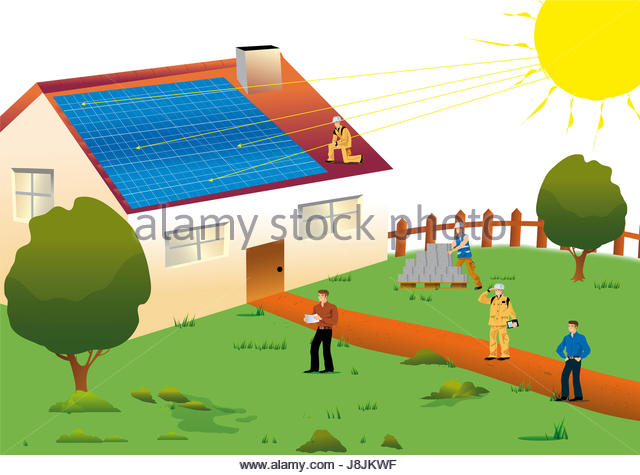In this animated clip art image, the setting features a house and a vibrant front yard. The house, depicted in a pinkish-white hue with an orange rust-colored roof, stands on the left side of the image. A large section of the roof is covered with blue solar panels. The sun shines brightly from the upper right corner, showcasing yellow rays, some of which transform into arrows pointing towards the solar panels.

A man, dressed in yellow with a white hard hat, kneels on the roof examining the solar panels. In the yard, two dark olive green trees frame the scene, one on each side of the image. The bright green grass, accentuated by tufts, forms a vivid front yard.

On the brown pathway that slices through the yard, two men are seen standing; one is clad in a long sleeve coat and pants, while the other sports jeans and a blue long-sleeve shirt. Another man, standing in front of this pathway, gazes at the tree while holding a paper; he wears a brown long-sleeve shirt with black pants.

In the background, a construction worker in a blue vest and brown pants is busy picking up cinder blocks or stones. Across the center of the image, 'Alamy Stock Photo' is superimposed in gray letters, indicating this depiction is a stock photo.